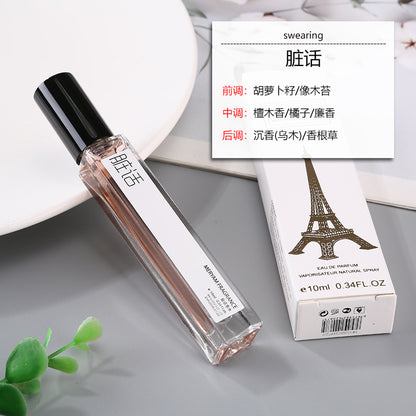The image is a detailed photograph of a perfume bottle, which is diagonally positioned with its black screw-on cap resting on the edge of a white ceramic plate. The bottle itself is made of glass, containing a pinkish or amber liquid. In the bottom left corner, there is a sprig of an artificial green plant, adding a touch of color and texture to the scene. 

To the right of the bottle, there is a white box, likely the packaging for the perfume, which bears the text "10 mL or 0.34 fl oz." The box also features a black illustration of the Eiffel Tower and includes a UPC code at the bottom. Overlaid in the top right corner of the image is a white text box with the word "Swearing" in black print, followed by Chinese characters. This text box has three lines, each beginning with two Chinese characters in red, a colon, and then more Chinese characters in black font.

The background surface that the plate and the bottle are on is a grayish countertop. The overall setting suggests an advertisement, with the detailed elements and layout emphasizing the aesthetic appeal and international flavor of the perfume.